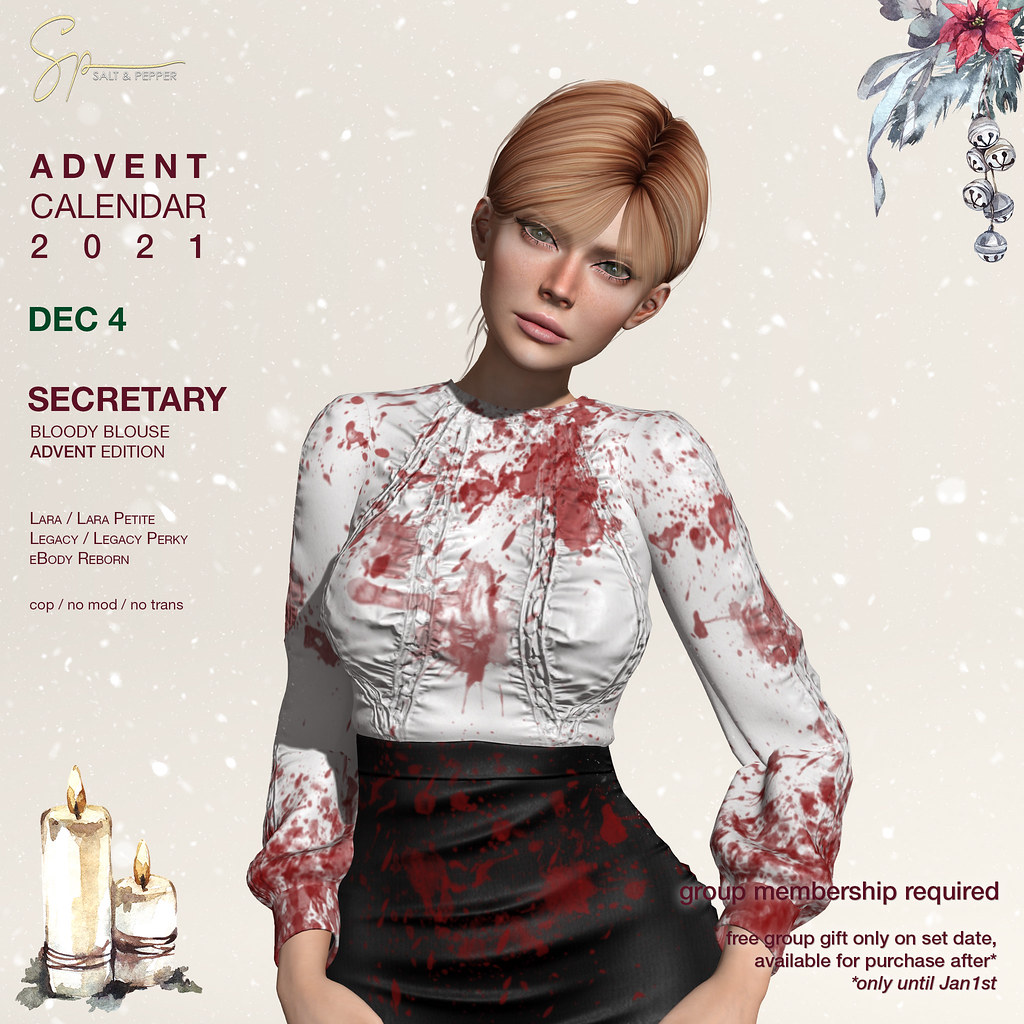This detailed illustration depicts a realistic, computer-generated image of a Caucasian woman with strawberry blonde hair and blue eyes, standing with her head slightly tilted. She is wearing an old-fashioned, white long-sleeved blouse that's splattered with what appears to be blood, lending a horrifying effect as it also stains her tight black skirt. The backdrop features a spotty beige and white pattern.

In the advertisement's text, on the left side, it is labeled "Salt-N-Pepper Advent Calendar 2021" with a specific focus on December 4th: "Secretary Bloody Blouse Advent Edition, Laura, Laura Petit. Legacy, Legacy Perky. E-Body Reborn. Cop, No Mod, No Trans." A striking pink flower with feathers and bells is illustrated at the top right. Below this, the text "Group Membership Required. Free group gift only on set day, available for purchase until January 1st" is displayed, clarifying the promotional details. On the bottom left, two candles are depicted, surrounded by leaves which add to the eerie, festive theme of the calendar ad.